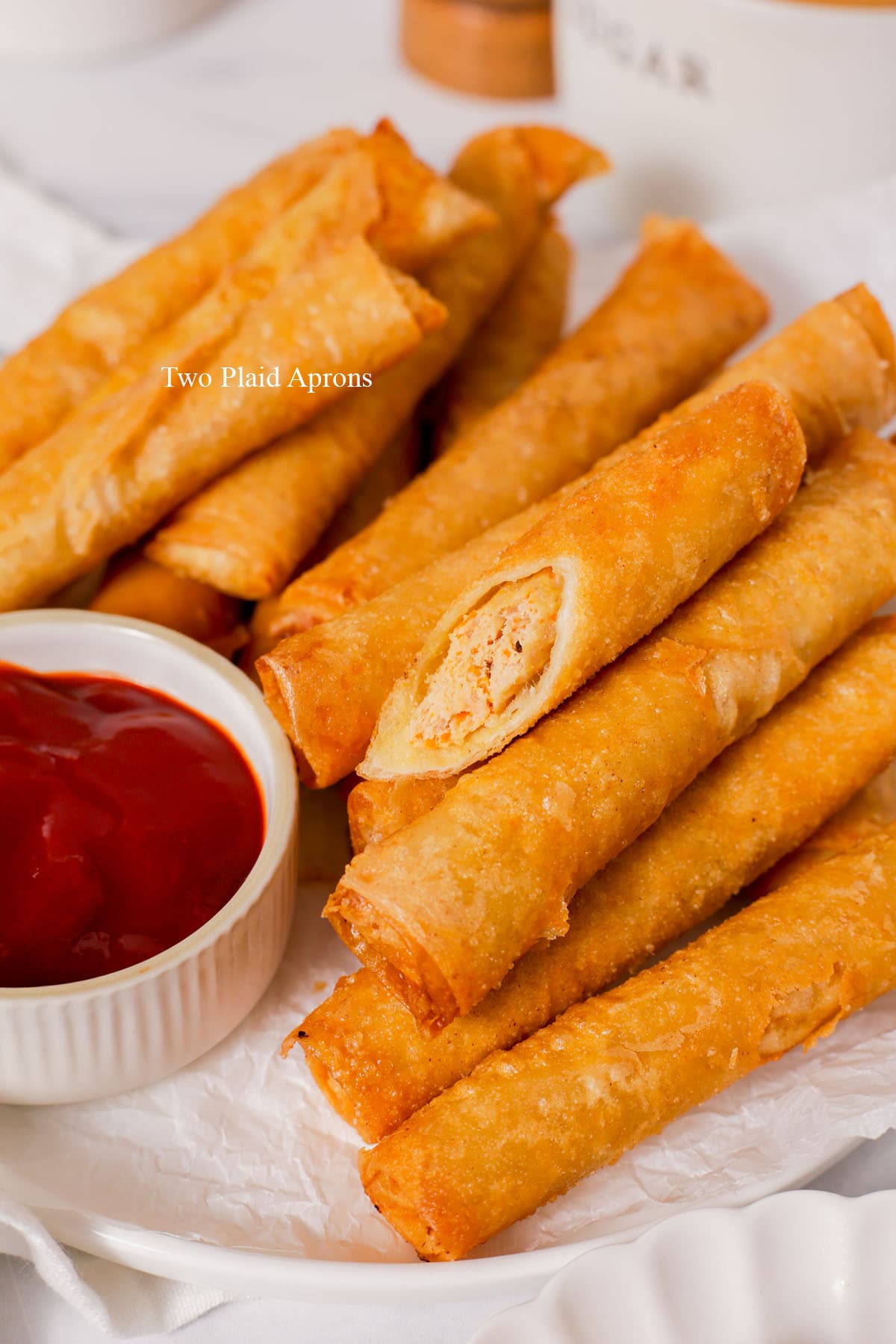This photograph features a delectable arrangement of savory egg rolls stacked haphazardly on a plate, overlaid on parchment or wax paper. The egg rolls, fried to a perfect golden brown, exude a crispy texture that contrasts beautifully with their doughy wrap and savory meaty filling. One of the egg rolls is cut diagonally, displaying its white and orange interior, which adds a peek into the delicious filling. On the plate, a small ribbed porcelain ramekin filled with a chili sauce or ketchup accompanies the egg rolls, positioned next to the food. The background of the image is clean and white, contributing to a food magazine or blog-like aesthetic. Another similar ribbed dish is visible at the bottom right of the image, completing this visually appealing and mouth-watering presentation.